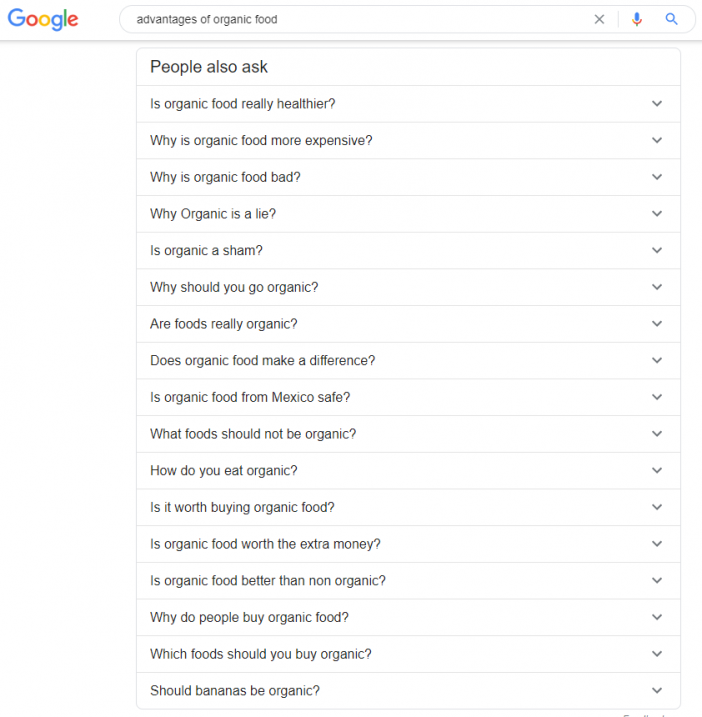The image is a screenshot of a Google search page displayed in light mode. In the top left corner, the recognizable Google logo is prominently featured. Below the logo, a search bar occupies the central part of the screen. To the right of the search bar, there is an 'X' icon, allowing users to clear any text they have entered. Adjacent to the 'X' icon, a microphone icon is present, indicating the functionality for voice input, where spoken words are transcribed into text. Additionally, a magnifying glass icon is shown, which users can click to initiate their search.

The search query displayed in the image is "advantages of organic food." Under the search bar, the "People also ask" section reveals various related questions posed by other users. These questions include:

- Is organic food really healthier?
- Why is organic food more expensive?
- Why is organic food bad?
- Why organic is a lie?
- Is organic a sham?
- Why should you go organic?
- Are foods really organic?
- Does organic food make a difference?
- Is organic food from Mexico safe?
- What foods should not be organic?
- How do you eat organic?
- Is it worth buying organic food?
- Is organic food worth the extra money?
- Is organic food better than non-organic?
- Why do people buy organic food?
- Which foods should you buy organic?
- Should bananas be organic?

These questions serve as suggested inquiries to help users further explore topics related to organic food. The screenshot emphasizes the use of Google in light mode, characterized by a predominantly white background.